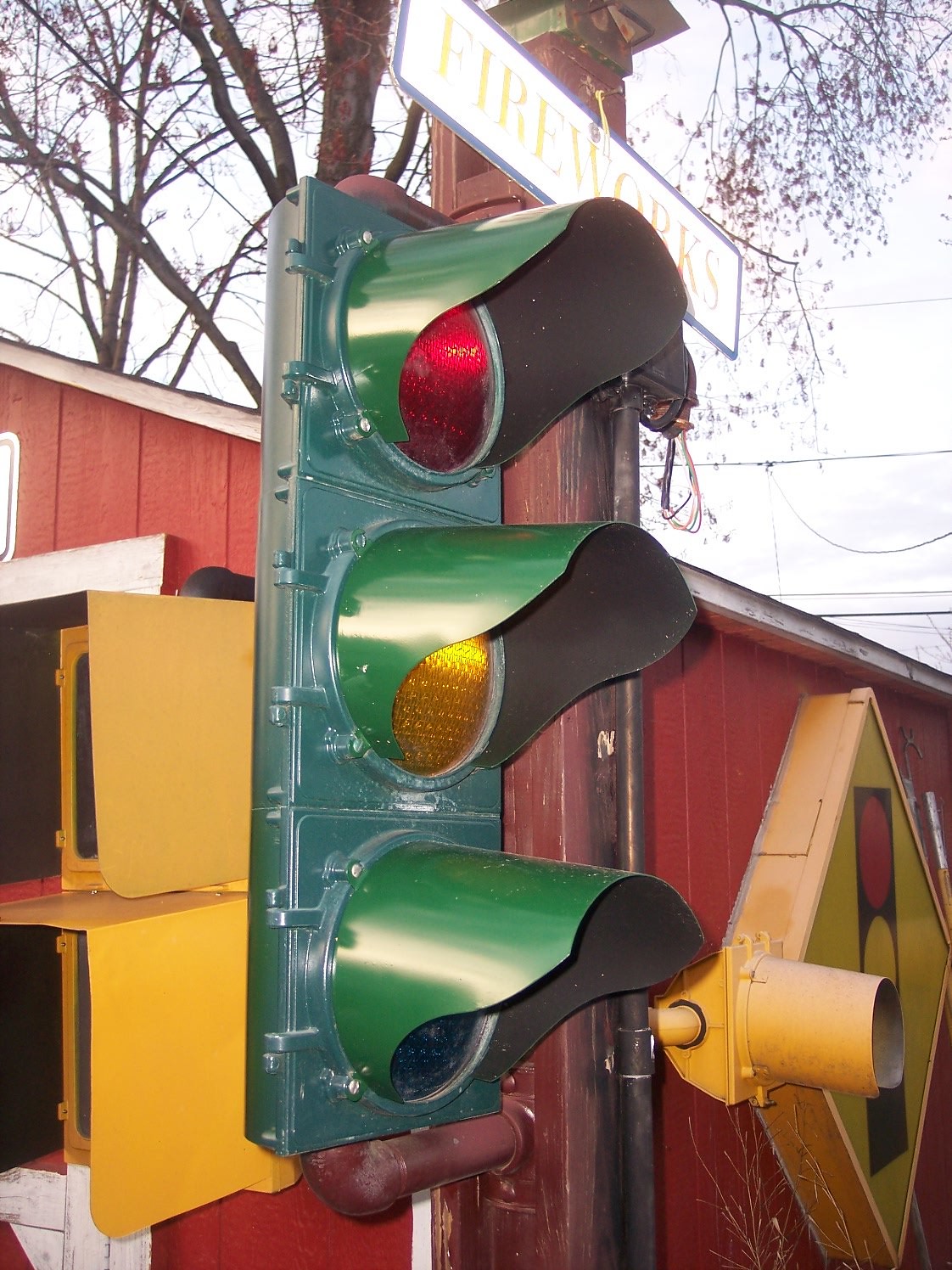An up-close photograph of a stoplight mounted on a wooden pole set outdoors under a light blue sky with a touch of trees in the top left corner. The central focus is the wooden pole, extending from the bottom to the top of the image. Atop the pole is a partially visible white sign that reads "fireworks." Affixed to the left side of the pole, and slightly closer to the camera, is a traditional stoplight with red, yellow, and green lights encased in green metal, mounted on a brown metal arm. Adjacent to this, on the backside of the pole, is another arm extending a triangular-shaped yellow sign featuring a black outlined depiction of a stoplight. Behind the main stoplight, two additional stoplights are slightly visible but partially off-screen. The setting appears to be near a red barn, visible from the door onward, with white trim and roofing, giving a rustic backdrop to the scene. In the background, a yellow sign adds another layer of detail, contributing to the ambiance that suggests a mix of utility and nostalgia. A glimpse of dark red fencing adds to the impression of a perhaps repurposed or cluttered yard area.